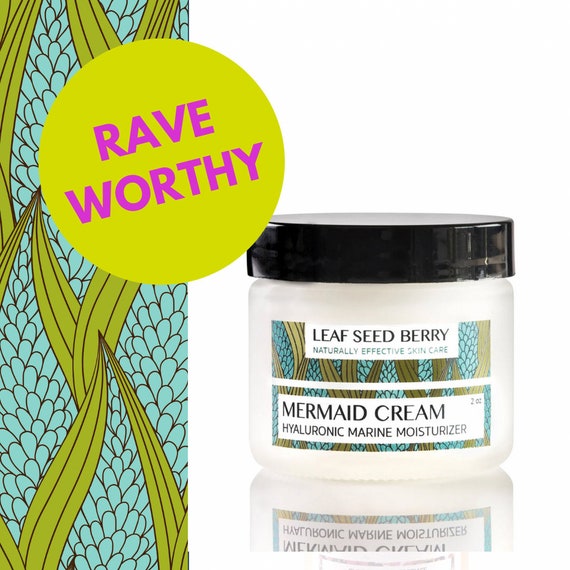The image is an advertisement for Hyaluronic Marine Moisturizer, branded as "Mermaid Cream" by Leaf Seed Berry. The scene features a clear, bright setting with a plain white background, focusing on a single jar of the cream, which is reflected on a glass surface below it. The product has a sleek black cap and a detailed label. The top part of the label prominently displays the brand name "Leaf Seed Berry" in capitalized black letters, followed by "Naturally Effective Skin Care" in blue, and "Mermaid Cream" in black. Below these, the product is described as "Hyaluronic Marine Moisturizer," also in black letters.

Accentuating the advertisement is a digitally added sign in the top left corner, which reads "Rave Worthy" in magenta-colored typography within a yellow neon circle. Additionally, a vertical banner with floral and leafy graphic designs runs along the left edge of the image. The combination of design elements, vibrant colors including teal, light green, light purple, off-white, black, and white, and clear, ample lighting make the product the undeniable focal point, effectively highlighting the cream's luxurious and naturally effective appeal.